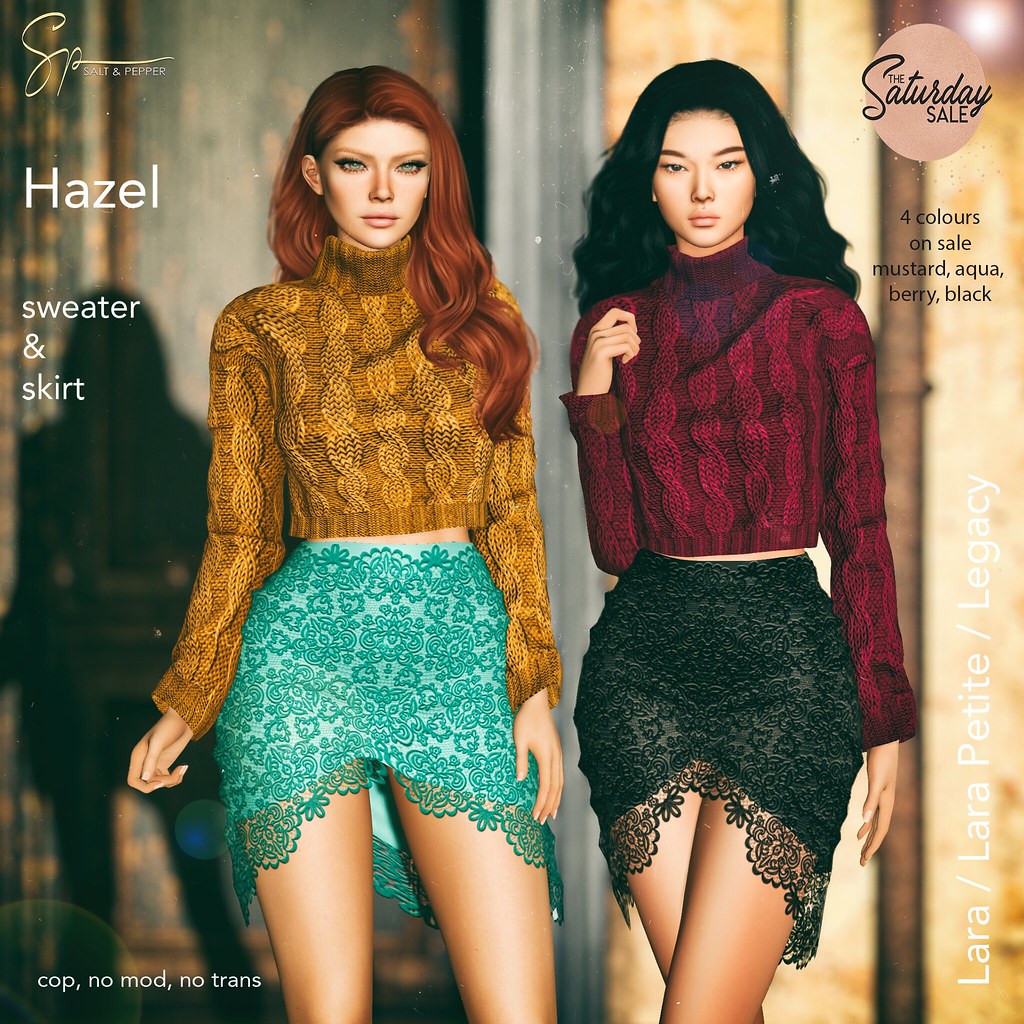The image is a detailed advertisement for a clothing sale featuring two highly realistic, CGI-rendered female avatars positioned at the center. Both avatars exhibit a sophisticated, modern style with distinct features: the avatar to the left has red, wavy hair and is dressed in a mustard-yellow sweater paired with an aqua lace skirt, while the avatar to the right has long, thick black hair and wears a berry-red sweater with a black lace skirt. Both avatars appear serious and stand against a backdrop that includes a large window, casting a shadow to the left of the red-haired avatar. The advertisement announces "The Saturday Sale," highlighting four colors on sale: mustard, aqua, berry, and black. Additional text includes "Lara, Lara Petite, Legacy, Hazel sweater and skirt," and sales conditions like "cop, nomad, no trans" suggest specific purchase terms. The ad's text is predominantly white and gold, with elements of gray and silver from the window in the background, contributing to an elegant and eye-catching presentation.